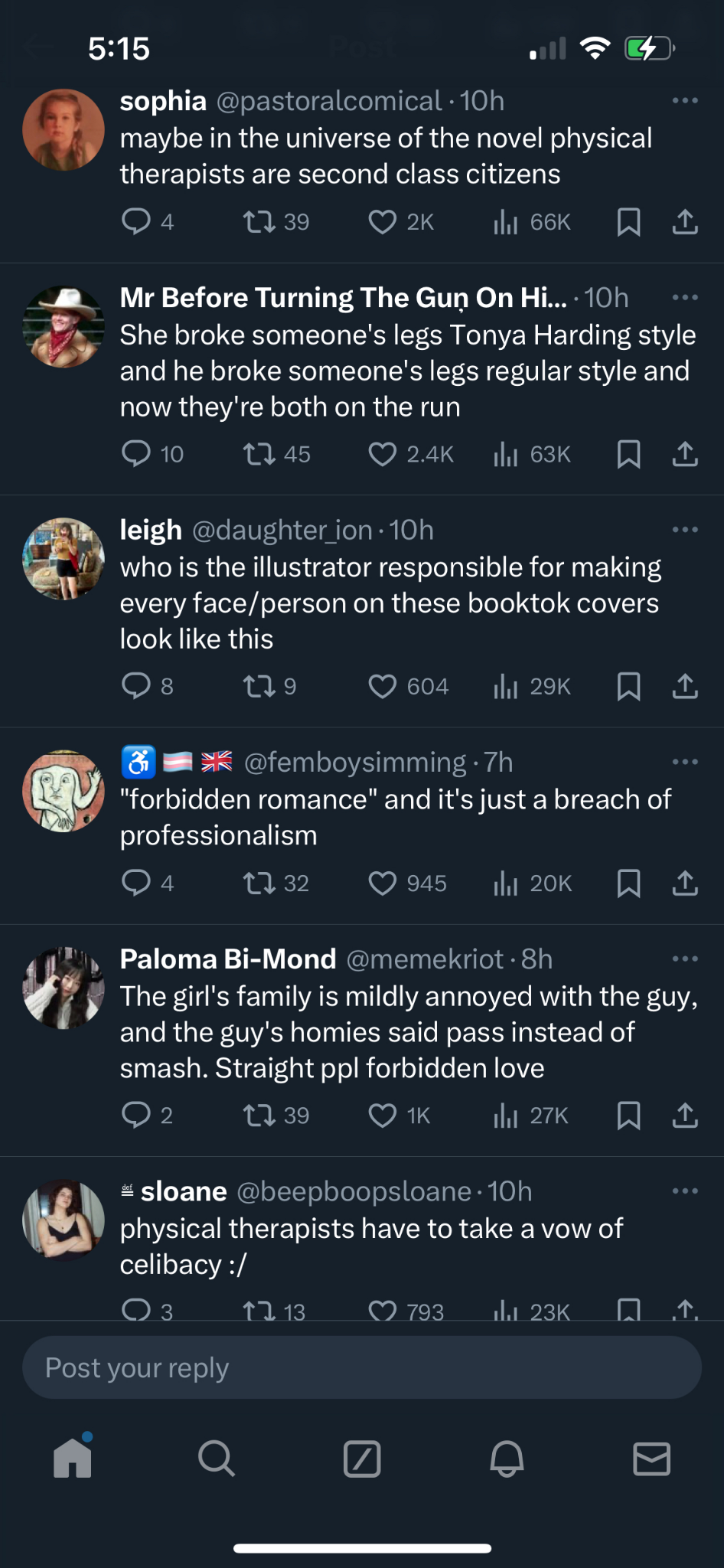**Detailed Caption for Screenshot:**

This image features a screenshot of a social media application with a predominantly black background. In the upper right-hand corner, a white numeral '515' is displayed, adjacent to icons symbolizing signal strength, Wi-Fi connectivity, and battery power, the latter of which indicates a level of around 50%.

The screenshot showcases six posts by various users. Each post is accompanied by the user's avatar on the left. On the right, the usernames are in bold white font. Directly adjacent to each username is their Twitter handle, formatted with an '@' symbol. The timestamp indicating how long ago each post was made follows the Twitter handle.

The posts are listed as follows:

1. The first post is by 'Sophia' (@PastoralComical) and was made 10 hours ago. The text of the post reads: "Maybe in the universe of the novel therapists are second-class citizens." Below this text, there are icons for commenting, retweeting, liking (represented by a white heart), views (noted as 66,000), and options for bookmarking or downloading the post.

2. The second post is by 'Mr. Before-Turning-the-Gun-On-Hit…' and states: "She broke someone's legs, Tonya Harding style, and he broke someone's legs regular style, and now they're both on the run."

3. The third post is from a user named 'Leigh' (L-E-I-G-H).

4. The fourth post features a username comprising various icons including the flag of Great Britain.

5. The fifth post is attributed to 'Paloma by dash Mond'.

6. The sixth and final post is by 'Sloane' (S-L-O-A-N-E) and reads: "Physical therapists have to take a vow of celibacy: /".

At the bottom of the screen, in a horizontal sequence, are icons for navigating the app: a home icon, search magnifying glass, a white square, a bell symbol, and an envelope icon. At the very bottom edge of the screen, there is a thin horizontal white line.

Overall, this detailed caption provides a comprehensive description of the screenshot, highlighting the content, user interface, and specific details of each post.